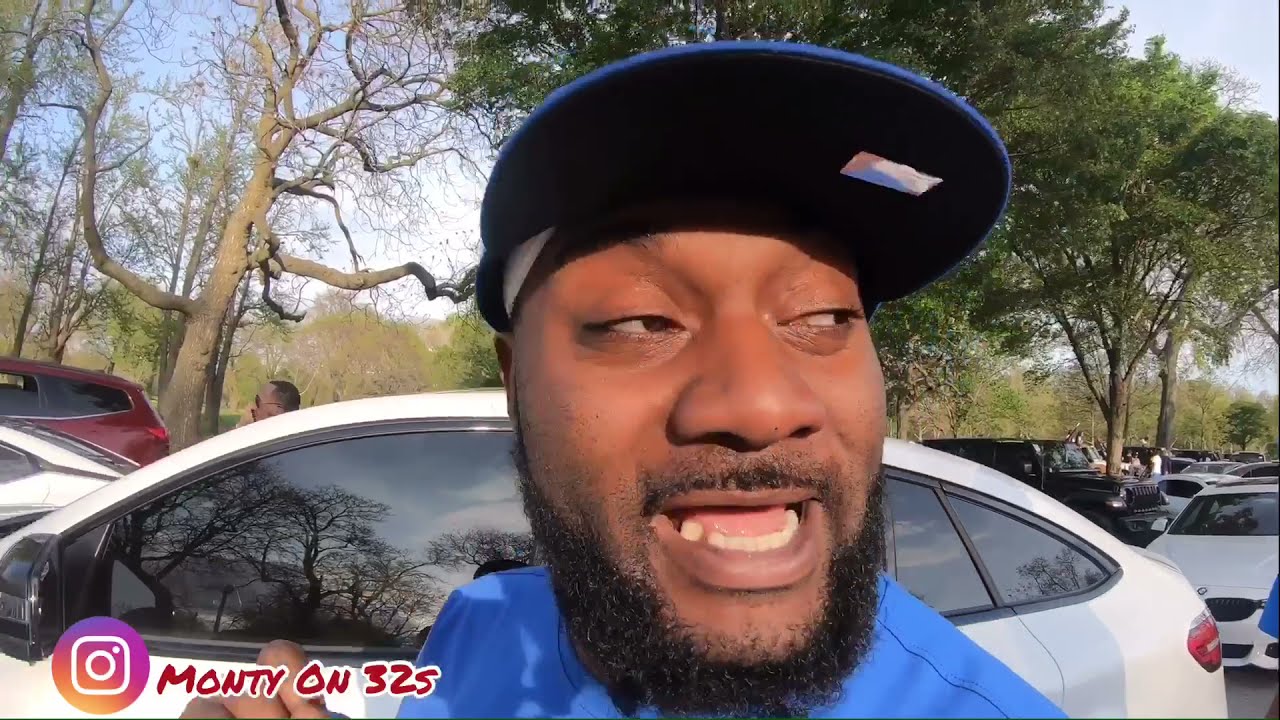In this image, we see a close-up of an African American man with a black beard, who appears to be speaking or shouting, as his mouth is open. He is wearing a blue and black flat-brimmed cap and a blue shirt. The man's gaze is directed to his right. Behind him, there is a white vehicle and a scenic backdrop featuring multiple trees; some trees are leafless, while others are lush with green foliage, suggesting a park-like setting. The sky above is a bright blue with scattered clouds, indicating it's daytime. In the lower left corner of the image, an Instagram handle is displayed in red text with a white border, alongside the Instagram logo and the phrase "Monty on 325." Additionally, there are several parked cars and people visible in the background.